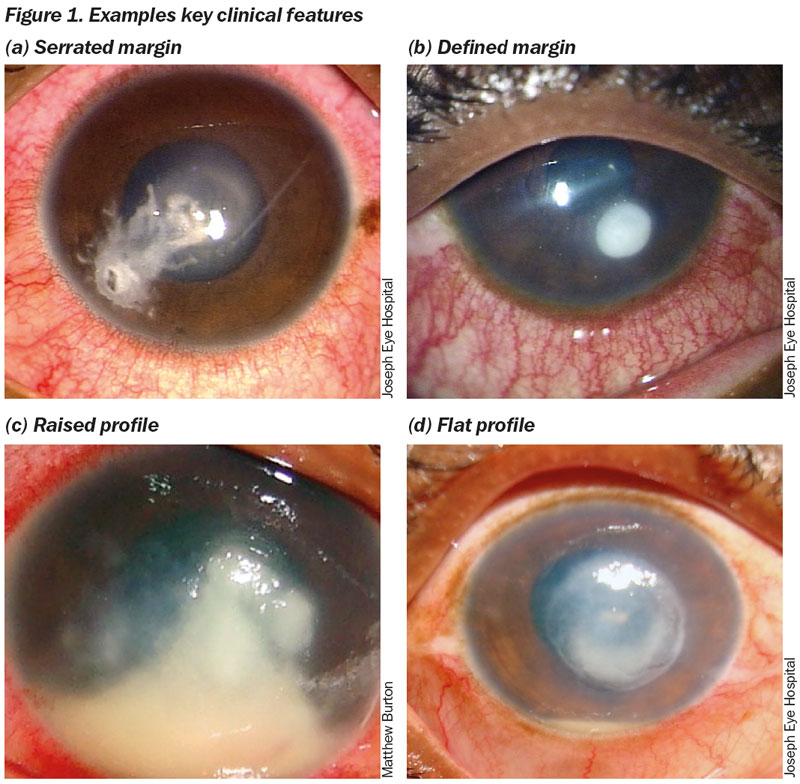The image is divided into four panels, each depicting an eye with noticeable abnormalities, labeled as "Figure 1 Examples: Key Clinical Features." The top-left panel, labeled "A, Serrated Margin," displays a brown eye with severe irritation. The eye is encircled by red veins, and a white, cloudy structure with a jellyfish-like appearance is evident at the bottom left, suggesting either an injury or illness. The top-right panel, labeled "B, Defined Margin," shows another brown eye with less pronounced redness but large red vessels. A distinct, circular white orb can be seen on the lower left portion of the iris, sourced from the Joseph Eye Hospital. The bottom-left panel, labeled "C, Raised Profile," presents an inflamed eye where almost the entire anterior iris is obscured by an uneven, white mass, indicating a severe condition. Lastly, the bottom-right panel, labeled "D, Flat Profile," features a brown eye with a conspicuous, circular white mass directly in the center of the pupil, suggesting a different yet significant ocular issue. Each image illustrates diverse clinical features of diseased or damaged eyes, emphasizing the severity and variety of these conditions.